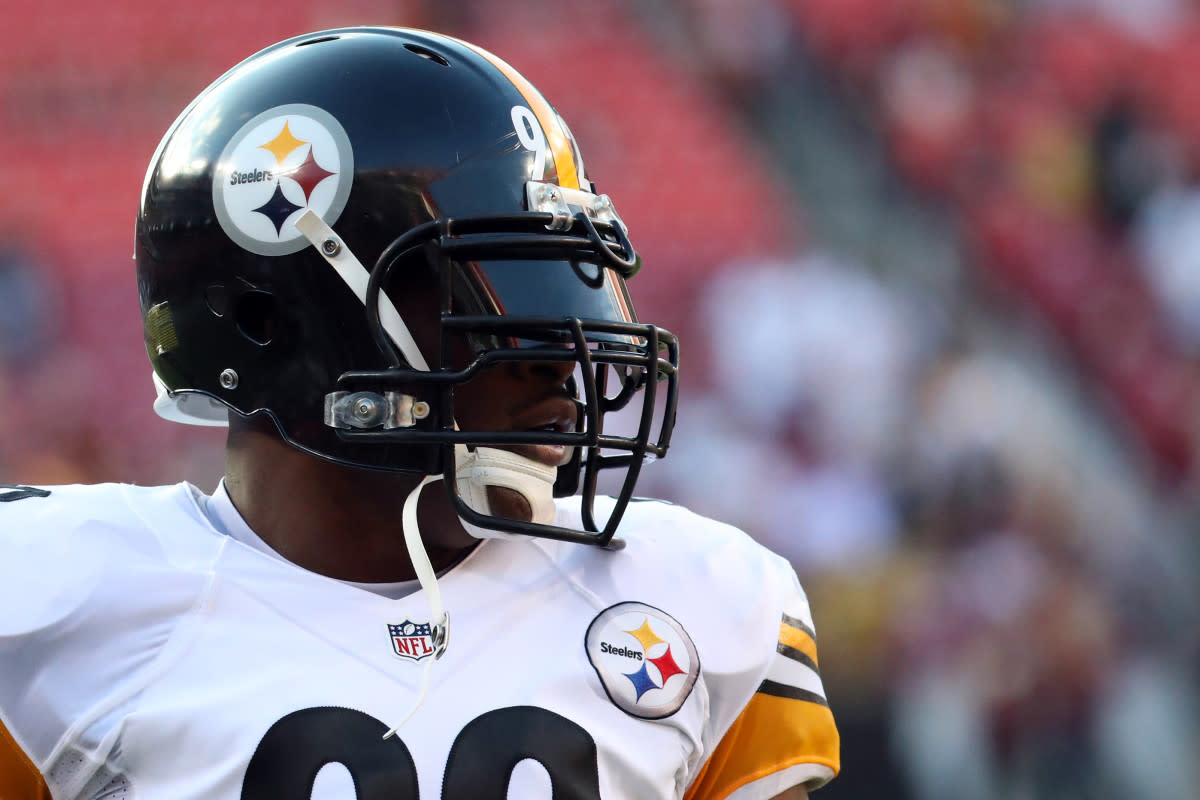This is a close-up portrait photograph of a Pittsburgh Steelers football player, an African American individual in full gear, focusing on his chest, shoulders, and helmet. He is wearing a black helmet with a prominent yellow stripe down the middle, and a circular white logo on the side that features the word "Steelers" in black letters accompanied by three four-point stars in blue, red, and yellow. A white stripe runs from the mouth area to the circular logo on the helmet. His helmet also includes a protective caged face mask and a black visor over the eyes. The player is turned slightly to his left, looking to his left, which is the right side of the frame. He dons a white jersey adorned with yellow accents on the shoulders and intricate stripes in black and yellow. The chest of the jersey bears an NFL emblem in red at the center, near the neckline, and another Steelers logo featuring the iconic three four-point stars outlined in blue, red, and yellow. The number 92 in white is partially visible on the top of the helmet next to the yellow stripe. The background includes blurred sand-colored stadium seats and red bleachers, keeping the focus on the player.